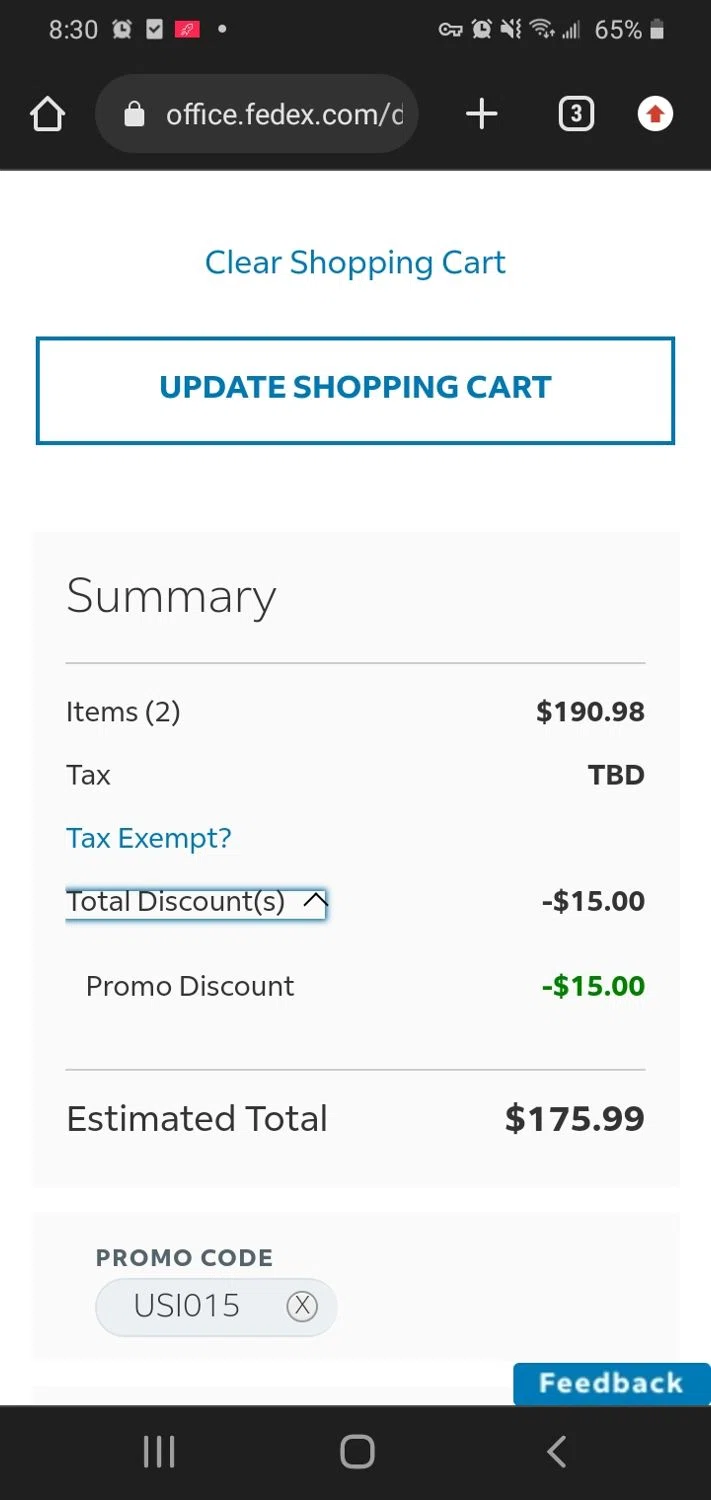The provided image is a highly stretched mobile screenshot, appearing edited with an exaggerated vertical elongation, particularly noticeable at the top.

### Header Section:
- The header features a black banner.
- Centrally placed in the banner is an address bar displaying "office.fedEx.com".
- On the top left, there's a home icon.
- To the right of the address bar, there is a plus icon, followed by a tab icon showing three open tabs.
- Further to the right, there is a white circle with a red star in the center.

### Body of the Web Page:
- The main body features a white background.
- At the top of this section, the text "Clear Shopping Cart" is prominently displayed in centered blue font.
- Below this, there is a large, horizontally stretched rectangle with a white background, containing the text "Update Shopping Cart" in bold blue print, centered within it.

### Summary Section:
- This section begins with a gray box labeled "Summary" in large gray letters at the top left.
- Below this label, a list of items is displayed on the left side, including:
  - Items
  - Tax
  - Tax Exempt
  - Total Discounts
  - Promo Discounts
  - Estimated Total
- Corresponding values listed on the right side include:
  - Taxes: To be determined
  - Discount: $15
  - Promo Discount: $15 (highlighted in green)
  - Estimated Total: $175.99

### Promo Code and Feedback:
- At the bottom, there is a thin gray box labeled "Promo Code" on the left.
- Next to this is a text box with numbers entered.
- The bottom right corner features a blue bar labeled "Feedback".

### Overall Description:
Despite being clearly edited with extreme stretching, this screenshot presents a detailed view of a shopping cart summary from the office.fedEx.com website, showing various elements of a typical checkout interface along with promotional discounts and a feedback option.